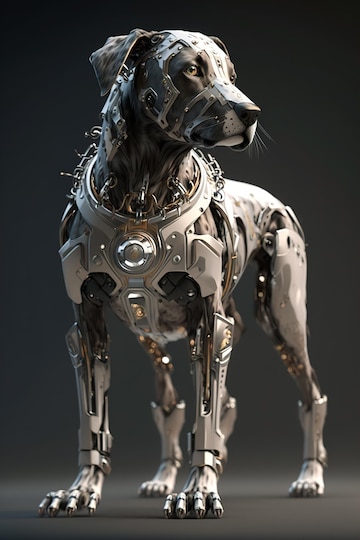This is a hyper-realistic digital creation of a black and white terrier dog, showcasing a fusion of organic and mechanical features. The dog is on all fours, looking off into the distance towards its left, set against a black gradient background. Its face and most of its upper body appear lifelike, but are interwoven with white and silver metallic armor that covers significant portions, including the face, chest, and legs. The dog's mechanical parts include entirely robotic legs, with visible wires extending to its body, accentuating a futuristic and somewhat robotic appearance. Details such as a white muzzle, black nose, spots on its floppy ears, and mechanical hands and feet contribute to its hybrid identity. Notably, the chest features a distinctive circular detail with a yellow crystal, potentially a source of light or an activation indicator. The image is of exceptionally high quality, with focused lighting that emphasizes the intricate details of the dog's mechanical and organic integration.